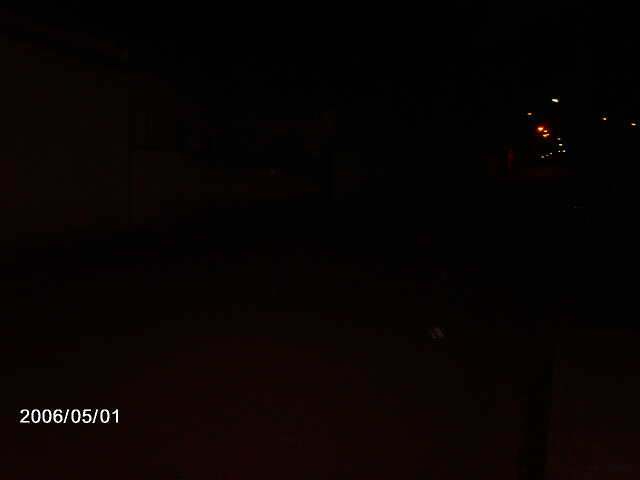This photograph, taken on May 1st, 2006, is predominantly a dark, blurred image with minimal visual detail. The date "2006-05-01" is visible in the bottom left corner. The rest of the photograph is mainly enveloped in blackness. However, a few scattered lights can be seen in the top right corner; these include red, yellowish, and small orange lights that resemble streetlights or city lights, offering a faint glimpse of illumination against the dark backdrop. The image gives an impression of being taken from a high vantage point, possibly from an airplane, looking down over a sparsely lit, rural area at night.